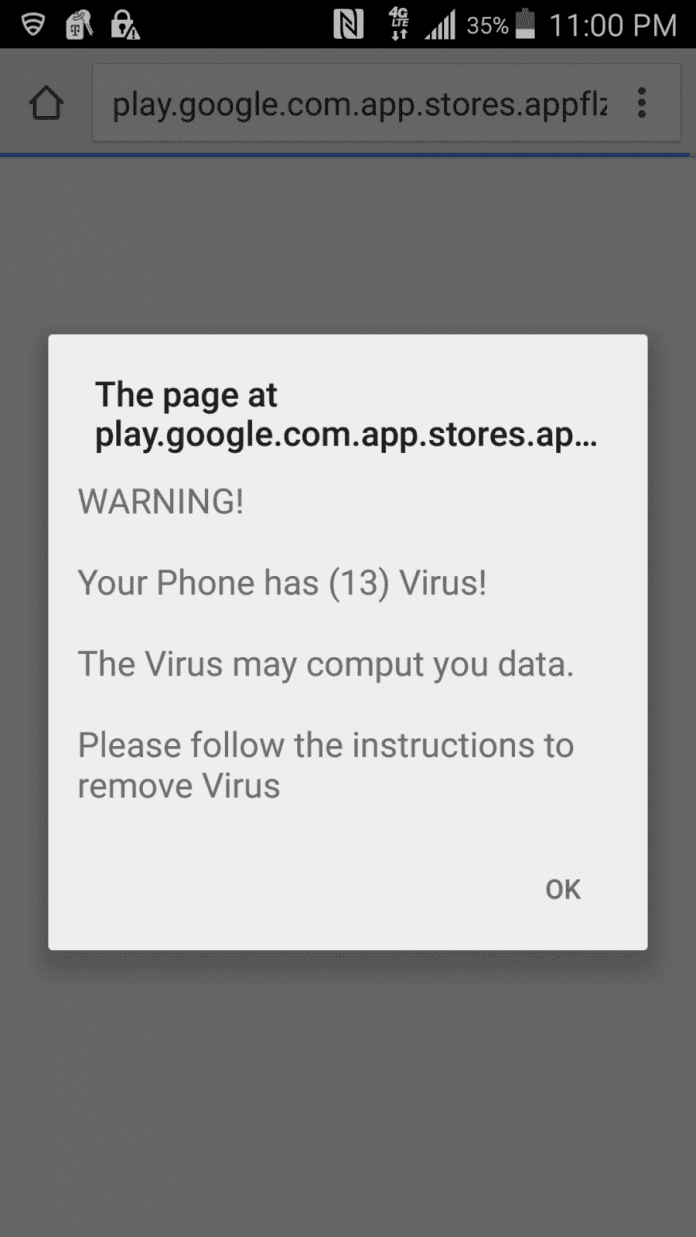The screenshot shows a deceptive popup on a smartphone browser with the URL partially visible as "play.google.com/app/stores/app.flz...". The popup warns the user with a message that begins, "The page at play.google.com/app/stores/ap... says: Warning! Your phone has (13) viruses!" It continues, "The virus may corrupt data. Please follow the instructions to remove the virus." The message is displayed within a white box featuring black text. At the bottom right corner of the popup, there is an "OK" button. 

The status bar at the top of the screen shows standard icons: signal bars, a padlock symbol indicating a secure connection, an NFC icon, 4G LTE signal, and the battery level at 35%. The time displayed is 11:00 PM, suggesting the phone might need charging soon.